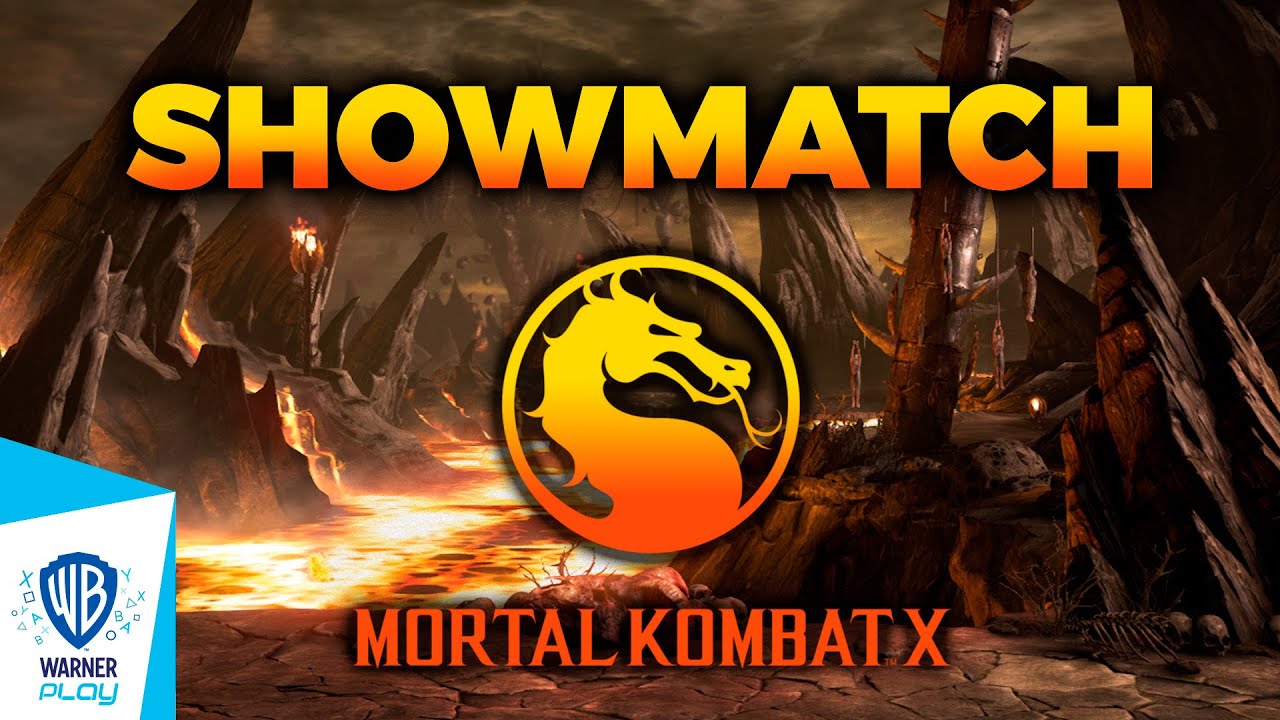The image is a detailed computer-generated ad for a show match of Mortal Kombat X. Central to the image is the iconic Mortal Kombat logo—a circular emblem featuring a dragon with a serpent-like tongue, with the top part of the emblem in yellow and fading to orange towards the bottom. The text "Show Match" appears at the top in a gradient from yellow to orange, while "Mortal Kombat X" is boldly displayed at the bottom in orange. In the bottom left corner, the blue and white Warner Play logo is visible, along with the familiar Warner Bros. emblem. The background is a menacing, dark scene reminiscent of a video game environment, featuring a dark gray, cloud-covered sky. Below this gloomy atmosphere is a vivid river of lava that starts at the bottom left and extends toward the center. Surrounding the lava are jagged, reddish rock formations jutting out at various angles, and lanterns filled with fire add to the infernal ambiance. Additionally, on the right side near the bottom, a skeleton can be seen among the rocks, enhancing the dark and foreboding nature of the scene.